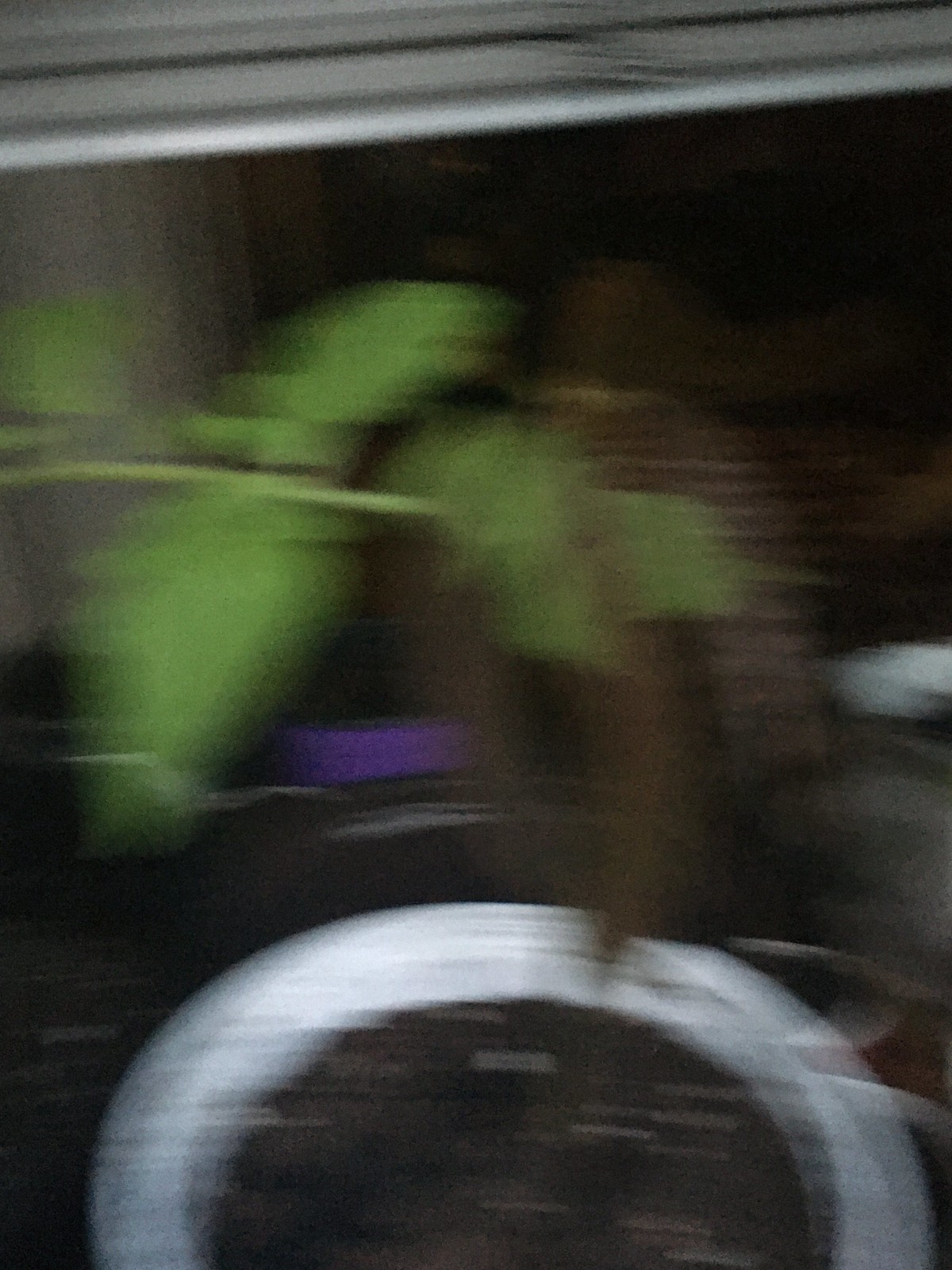This is a very blurry and out-of-focus photograph depicting a potted plant. At the bottom of the image is a circular white pot, possibly ceramic or plastic, filled with brown soil. A single stem with clusters of leaves rises from the center of the pot. The leaves are primarily bright green, with some exhibiting a variegated maroonish coloration. Surrounding the pot and plant, the background consists of obscure brown, tan, and grayish objects, making it difficult to distinguish specific details. The upper right corner of the image appears darker, and there is a subtle suggestion of a metallic beam at the very top of the frame.